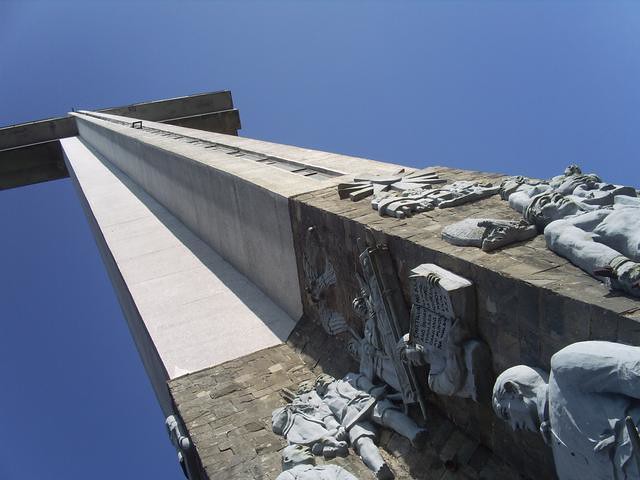The image captures the view from the bottom looking vertically upwards and slightly to the left at a monumental tower. This tower is composed of square beams primarily made of gray concrete, with the beams at the top extending outwards to form a T shape. Gray statues of people adorn the lower section of the tower, arranged around a base of intricately designed bricks, which appear to be fashioned from rocks. Notably, a man with combed-back hair gazes downward from the lower right side, and above him, a sculpted open book with black lettering is prominently displayed. The tower also features a sundial, or possibly a windmill sculpture, situated above the figures. Handles can be seen protruding from the top center beam, adding an additional layer of detail. The entire scene is set against a perfectly clear blue sky, which forms the backdrop for this detailed and dramatic architectural and sculptural composition.